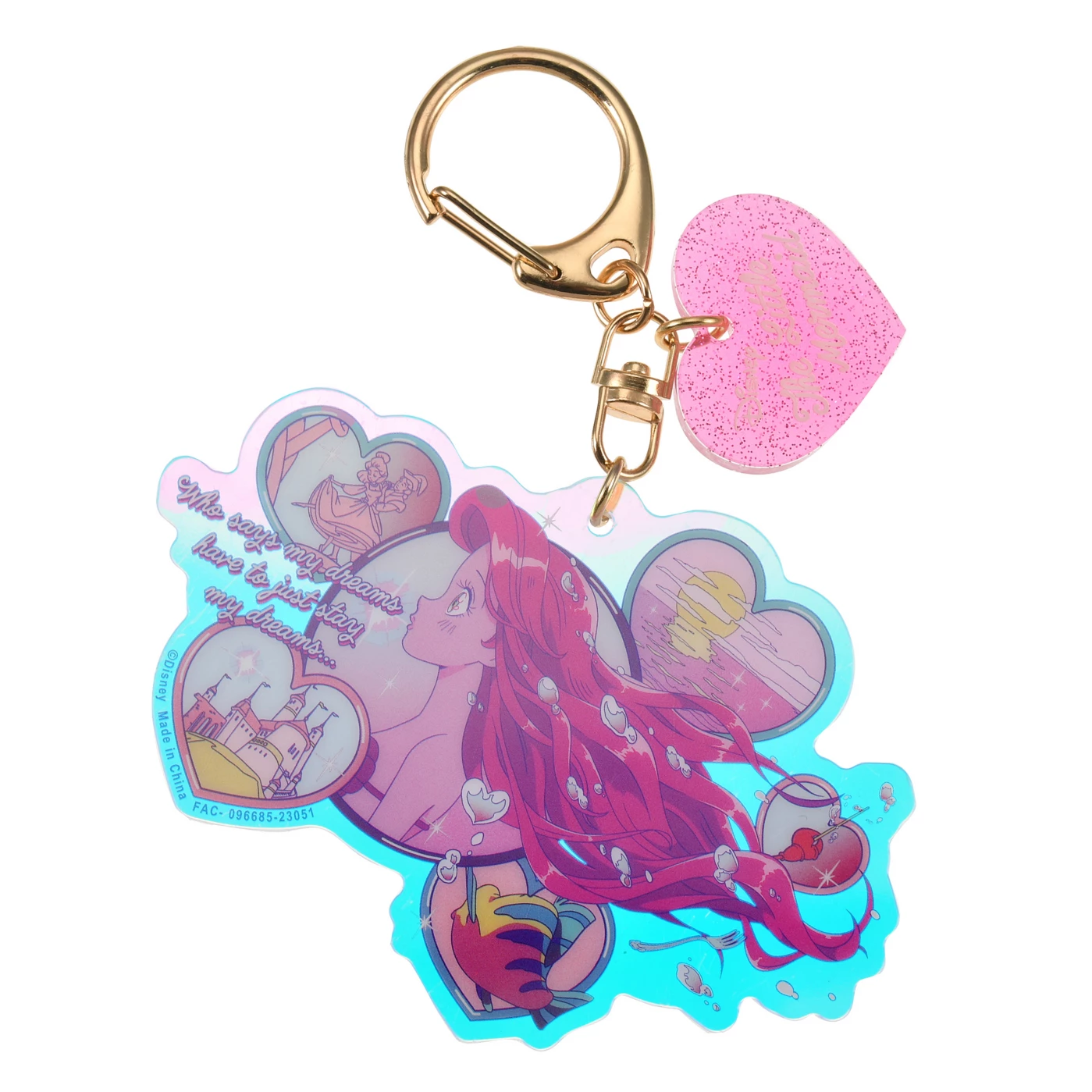This product listing image showcases a Disney-themed keychain against a white background. The keychain features a gold-colored, flat rectangular bar clasp attached to a gold chain. The main part of the keychain is crafted from an iridescent pink and blue plastic, shaped to frame various scenes from "The Little Mermaid" within heart-shaped insets. Central to the design is a circular encasing featuring Ariel with her flowing red hair and shell bikini top. Surrounding her are heart-shaped images: a castle, a sunset over water, Flounder, and Sebastian. Additionally, a detached pink heart with purple glitter dangles from the chain, bearing the text "Who says my dreams have to just stay my dreams?" On the left side of the main keychain, the same inspirational phrase is written. The bottom edge of the keychain notes "Copyright Disney, Made in China, FAC 096685-23051."